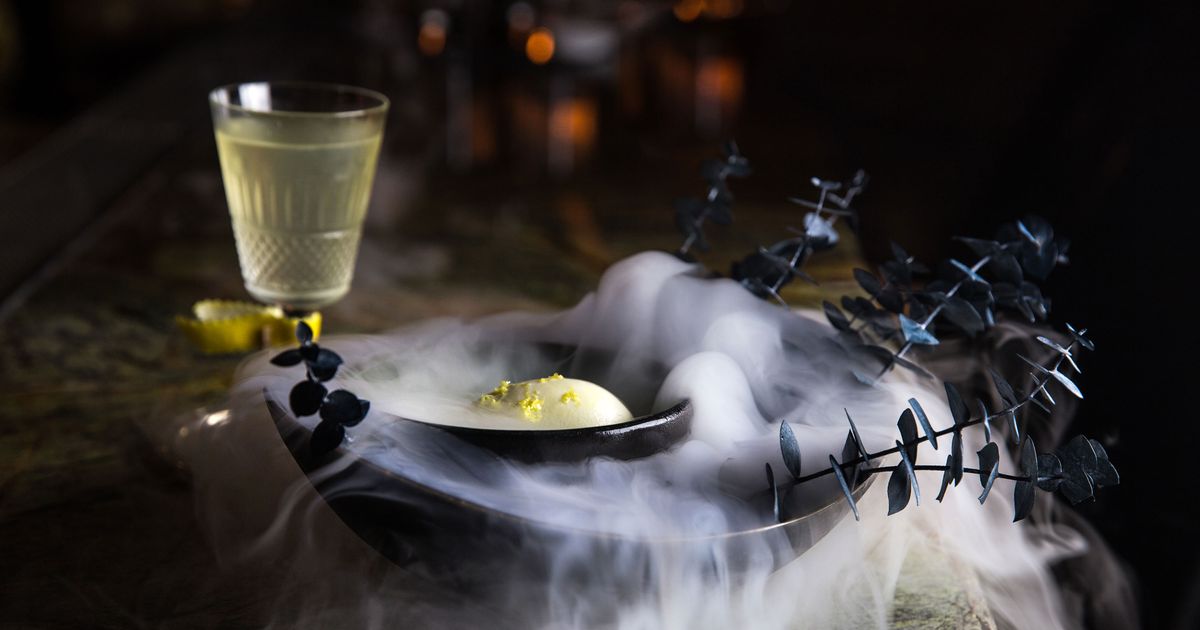The image showcases a dramatic culinary presentation centered around a steaming cauldron-like bowl, from which thick, white smoke, possibly from dry ice, billows out, creating a mystical ambiance. Within this large bowl sits a smaller pan or skillet containing a white substance that resembles dough or ice cream, speckled with yellow seasoning or crumbles. Decorating the right side of the bowl are dark green leaves, possibly for garnish, adding a touch of natural elegance. Flanking this elaborate setup is a clear glass filled with a light beige liquid, possibly juice or wine, enhancing the sophisticated and intriguing nature of the scene. The entire arrangement rests on a marble countertop, with a blurred, indistinct background that places full focus on the culinary display.